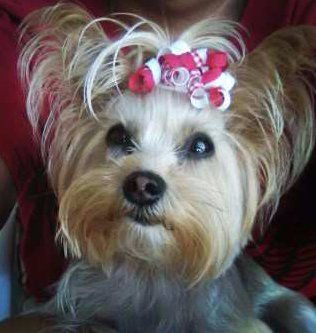This is a close-up headshot of an adorable Yorkie with long, fluffy hair styled around its face. The Yorkie's large black eyes and black nose are prominent features, and its mouth is closed. The dog sports a decorative, curled ribbon in its hair, which is a mix of red and white colors. Its face is mostly lighter brown, with darker brown fur resembling a mustache on the sides of its nose. Behind the ribbon, some strands of its hair appear white, transitioning into darker brown and gray around the neck. The background behind the Yorkie is a blend of black and red, adding to the contrast. The dog, which appears female due to the ribbon, is posing and looking directly at the camera, making it the focal point of the image. The photo captures the Yorkie's fluffy, wispy hair and detailed ribbon, providing a charming and detailed portrayal.